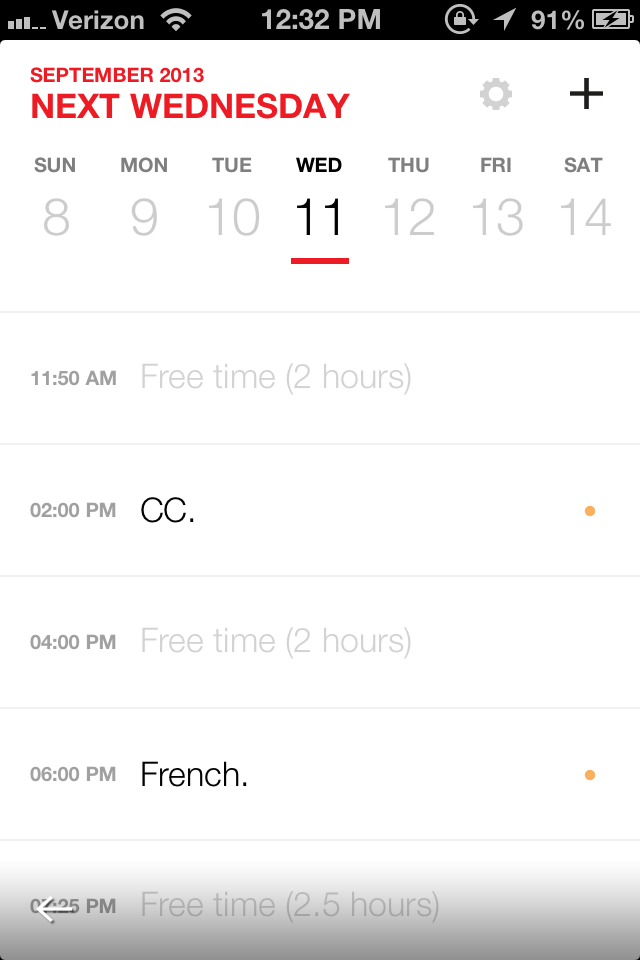This image shows a smartphone screen displaying a scheduling or calendar application. 

At the very top of the screen is a black status bar. On the left side of this bar, there are three signal bars, with the middle two signal bars filled, indicating signal strength. To the right of these bars, the word "Verizon" is displayed in white text. Next to “Verizon,” there is the signal icon, followed by the current time, "12:32 p.m.," also in white text. There is also a padlock with an arrow circling around it, indicating screen orientation lock. Further to the right, an arrow points to the right, followed by the battery icon which displays "91%" and indicates that the battery is charging, as shown by the charge symbol in the center of the battery icon.

Beneath the status bar, in red text, the date "September 2013" and the text "NEXT WEDNESDAY" (capitalized) are displayed. To the right, there are icons: a circle with a gear symbol and a black plus sign.

The weekdays are listed below in gray text: "Sunday," "Monday," "Tuesday," and "Thursday" to "Saturday." "Wednesday" is highlighted in black text. Under this, the dates are shown in gray text, except for the 11th, which is highlighted in black with a red underline.

Further down, a gray horizontal line divides the date section from the schedule. At 11:50 a.m., there is a gray text entry showing "Free time - two hours" (with "two hours" in parentheses). Below that, there is a 2 p.m. entry labeled "CC." To the far right of this entry, there is a small orange circle. 

At 4 p.m., "Free time - two hours" is noted again, with "two hours" in parentheses. Then at 6 p.m., the text "French." is displayed in black text, followed by an orange circle at the far right. 

At the bottom of the screen, half-covered by a white arrow pointing left, the time and "Free time - two and a half hours" (with "two and a half hours" in parentheses) are partially visible.